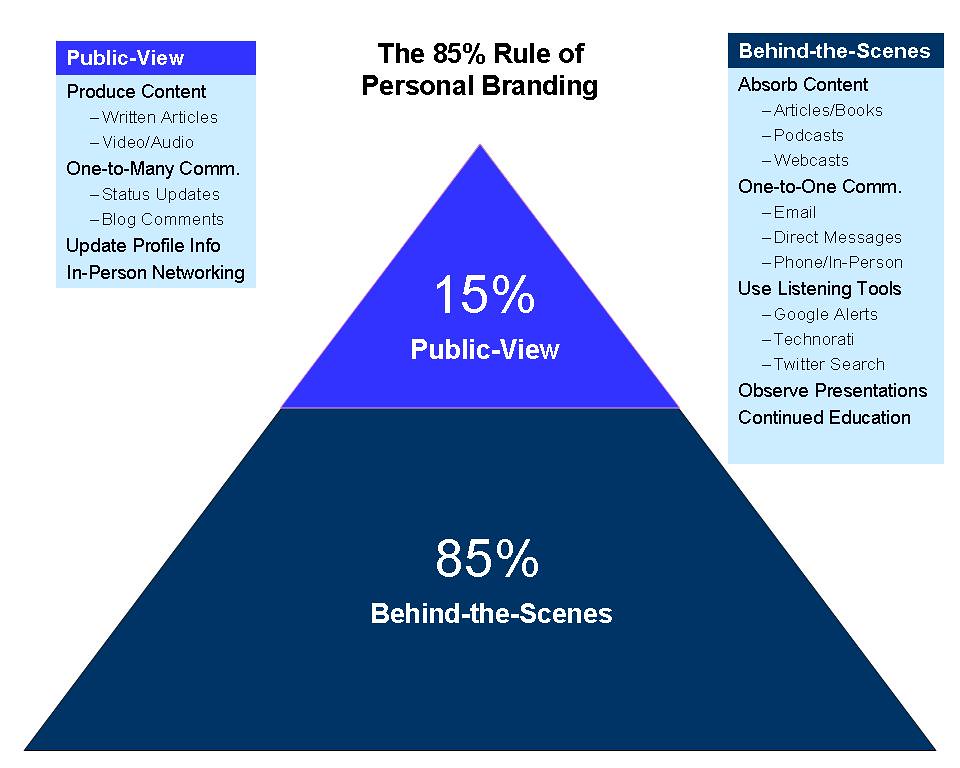Introducing the "85% Rule of Personal Branding" infographic, designed as a visually appealing training PowerPoint slide. Set against a clean, white background, the central focus is a triangle divided into two sections: the top 15% in bright blue, labeled "Public View," and the remaining 85% in a darker blue, labeled "Behind the Scenes."

Above the triangle, the main title reads, "The 85% Rule of Personal Branding." Flanking the triangle are two detailed vertical columns. 

The left column, titled "Public View," lists methods for outward engagement:
- Produce Content
- Written Articles
- Video/Audio
- One-to-Many Communication
- Status Updates
- Blog Comments
- Update Profile Info
- In-Person Networking

The right column, titled "Behind the Scenes," outlines practices for internal development and observation:
- Absorb Content
- Articles and Books
- Podcasts
- Webcasts
- One-to-One Communication
- Email
- Direct Messages
- Phone
- In-Person
- Use Listening Tools
- Google Alerts
- Technorati
- Twitter Search
- Observe Presentations
- Continued Education

This comprehensive graphic highlights the significant disparity between public visibility and the private efforts that support a robust personal brand.